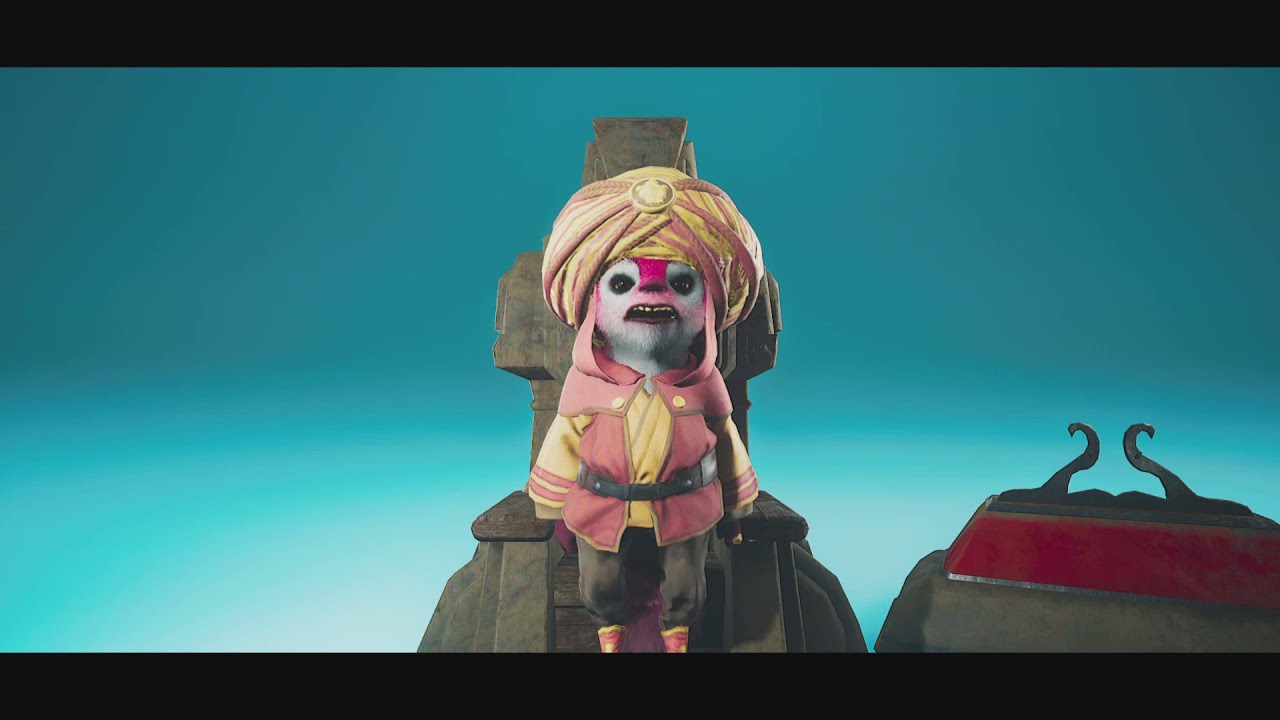The image depicts a computer-generated cartoon character, likely a stuffed animal or doll-like figure. This furry creature is adorned with a large yellow turban featuring pink outlines, which extends down to its elaborate pink and yellow jacket that resembles a pirate coat. A belt cinches the coat at the waist. The character wears baggy brown pants tucked into sharp pink boots. Its face is characterized by human-like eyes, a pink nose that runs down its forehead attached by a pink strap, and visible upper teeth. The background consists of an ancient ruin with a grainy blue sky that lightens towards the bottom and is bordered by black letterboxes. To the right, there is a stone statue and a scroll-like gray object sticking up, alongside a velvet-like red wedge shape. The character appears to be leaning or sitting on what looks like a stone throne.